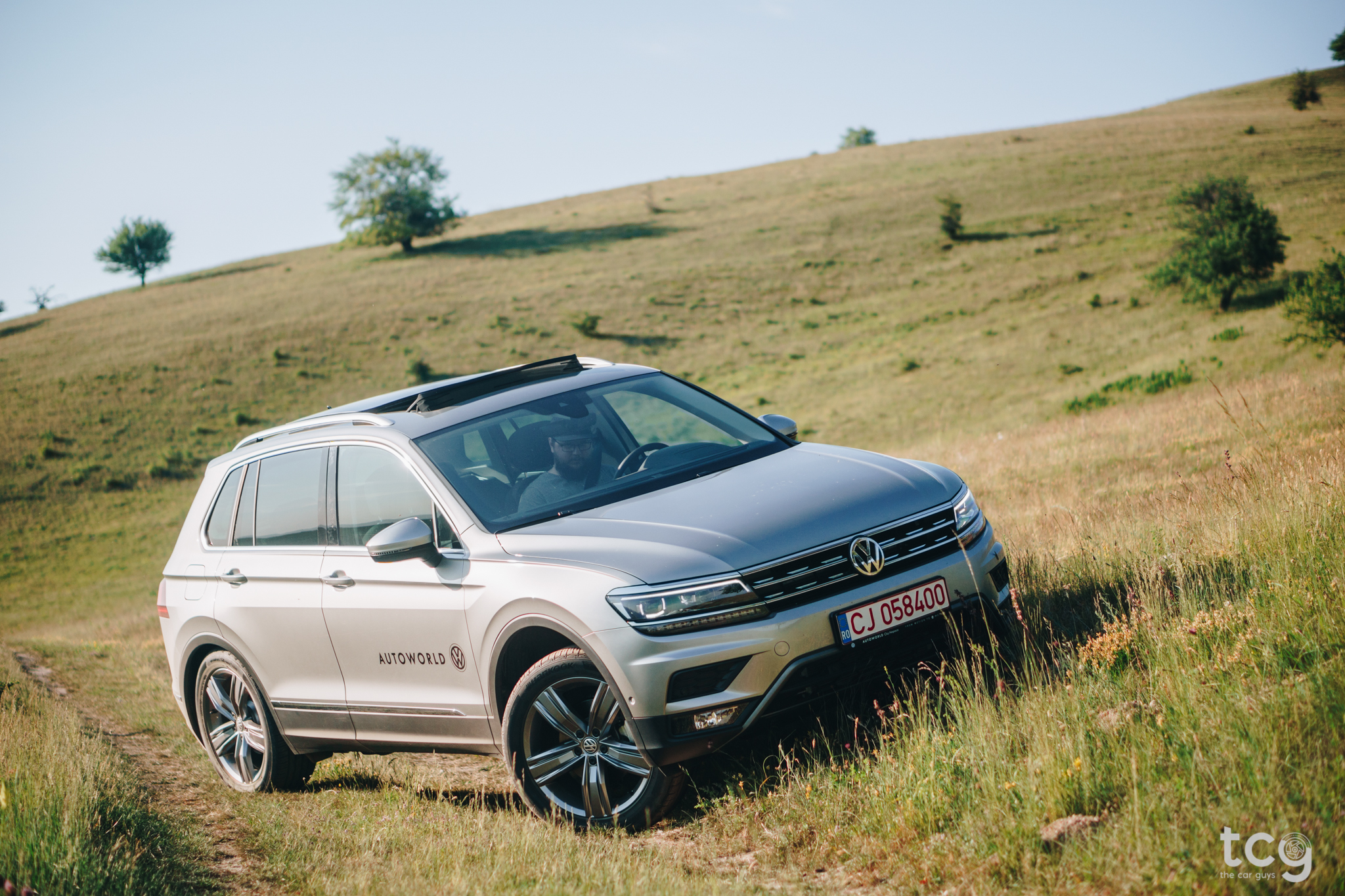In this close-up, angled photograph, a silver Volkswagen SUV with four doors is parked on a grassy hillside. The vehicle is seen from the front-right side, showcasing the prominent Volkswagen logo centered on the front grille. The front right wheel is turned slightly, and the car's sunroof is partially open with tinted windows. The sedan sits on a sloped hill, with the left set of wheels positioned higher than the right. Surrounding the vehicle is a dried tan grassy field with patches of green grass and scattered trees, including some in the foreground and on the left side of the image. In the background, the landscape features rolling hills and additional trees. The vehicle's license plate is a long, rectangular European style with a black outline and red lettering. Inside the SUV, a bearded man is visible behind the steering wheel. The ornate hubcaps feature five-petal designs. The image also includes a watermark in the lower right corner that reads "TCG" or "TCY". The photo captures a tranquil, natural environment under a blue sky, with no additional text aside from the watermark and logos. In the corners of the image, there are also noticeable areas of tall grass and weeds.